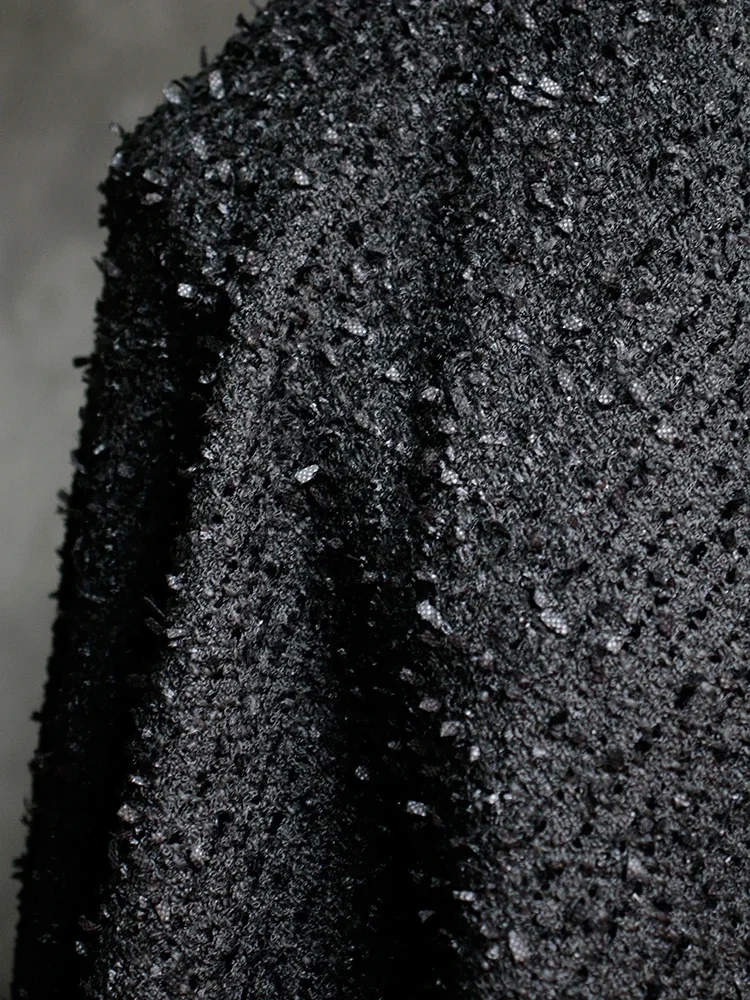The image showcases a highly detailed, close-up view of a textured black fabric, which appears to be part of a sweater or jacket. The fabric is predominantly black with intricate weaving that creates a textured effect, reminiscent of a Chanel suit. The material features both horizontal and vertical lines—horizontal lines along the main body and vertical lines along what seems to be the arm—adding dimensionality to the fabric. Additionally, there are small flecks of material scattered across the surface, some of which appear lighter, likely due to the way the light highlights them. These flecks contribute to the rough texture of the fabric. The light playing on the surface also gives certain areas a shimmery appearance, possibly making those sections look like recycled plastic. The background is a dark gray with lighter patches, enhancing the contrast and emphasizing the fabric's detailed texture.